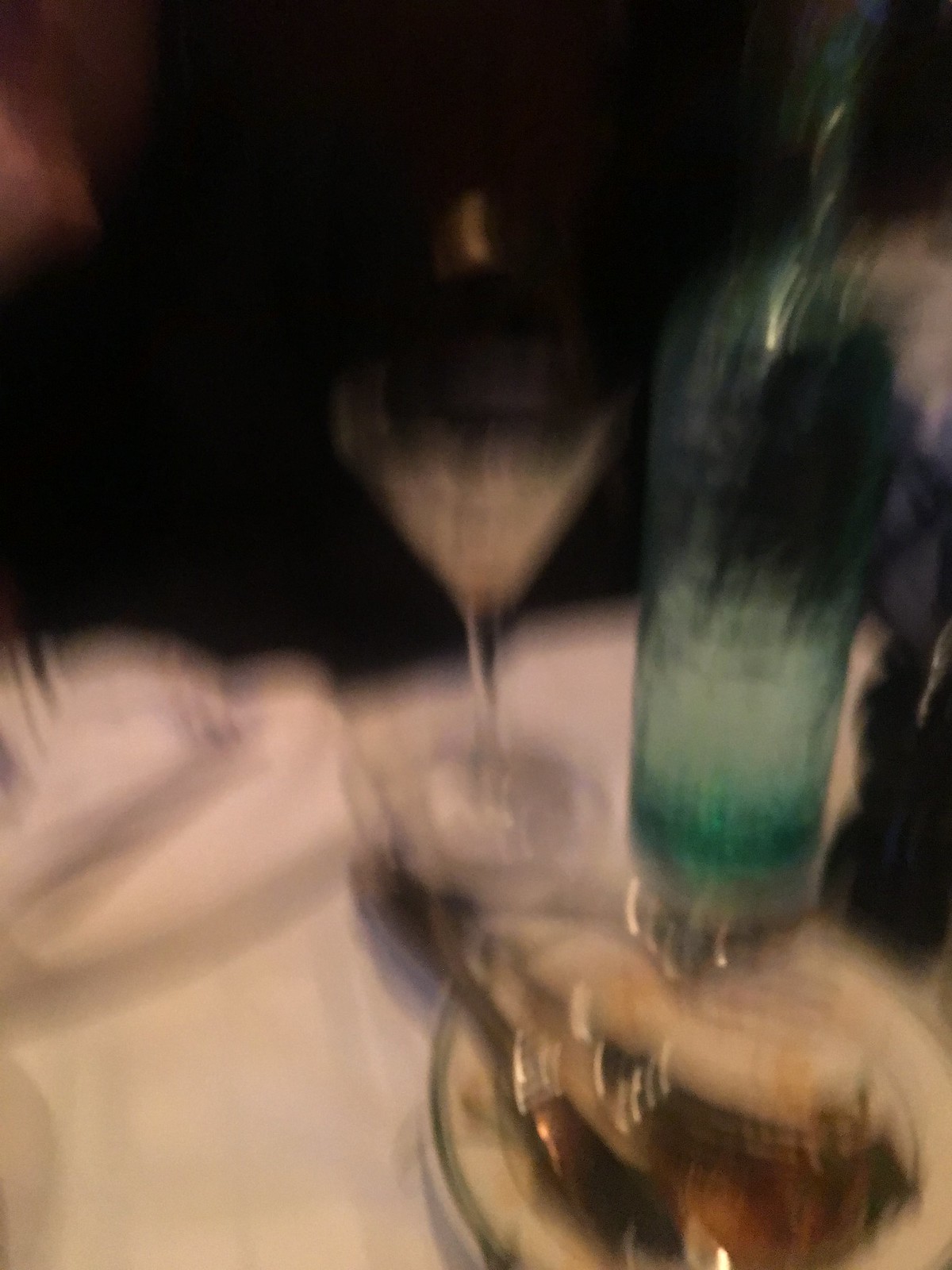The image depicts an extremely blurry scene of a dining table at a restaurant. The table is covered with a white tablecloth, creating a stark contrast with the dark upper background. On the table, there is a small white plate that appears to be almost empty, save for a few remnants of possibly half-eaten food. The plate is accompanied by a couple of forks lying on it. Toward the center, there is a clear cocktail glass partially filled with a yellowish drink, and nearby, a clear green cylindrical bottle, likely a wine bottle, which still has some liquid inside. Additionally, there's a white, possibly used, folded napkin situated beside the glass. The overall scene suggests the remnants of a recently finished meal, but the significant blurriness of the photograph makes it difficult to discern finer details.